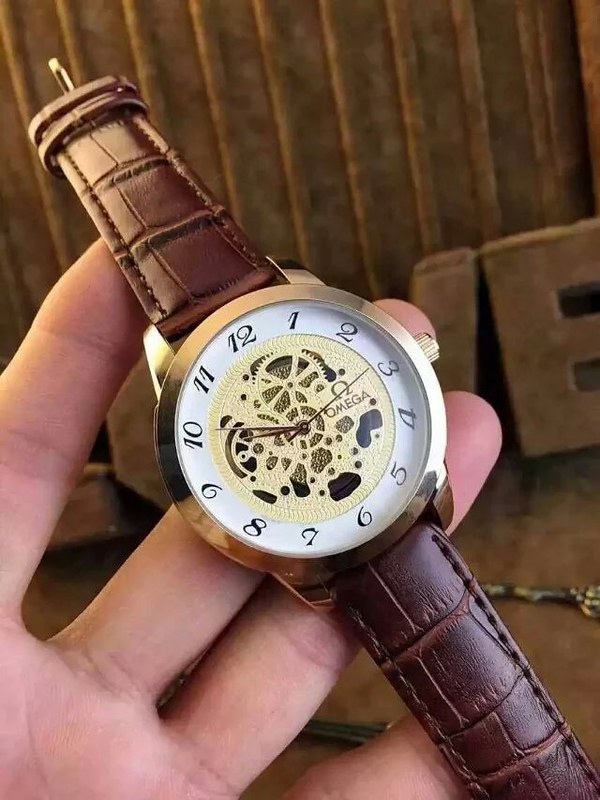In the photograph, a person's left hand extends into the frame from the bottom left corner, holding up a wristwatch at an angle that runs diagonally from the lower right to the upper left corner. The fingers are positioned such that the index finger is spread slightly away from the middle and ring fingers, which are together, while the pinky is extended further out. The palm is slightly visible below the ring finger, and the fingertips are subtly positioned behind the watch, providing support. The watch's band is a textured brown leather that resembles crocodile skin, though it is likely just a pattern and not genuine leather. The frame of the wristwatch is gold, with a matching gold crown for adjusting the time located on the right side of the case. The outer edge of the watch face is also gold, encasing a white dial featuring black numbers 1 through 12 in a traditional arrangement. Inside the white dial is another gold-bordered section that reveals the intricate gears and inner workings of the watch. The watch features two thicker hands, one short and one long, as well as a thin second hand. The name "Omega" is inscribed in black lettering on the right side of the dial near the 3 and 4 o'clock positions. The background includes a wooden wall with partial lettering visible between the fingers, including parts of the letters "L," "O," "V," and a full "E," suggesting some kind of sign or word against the brown ground.